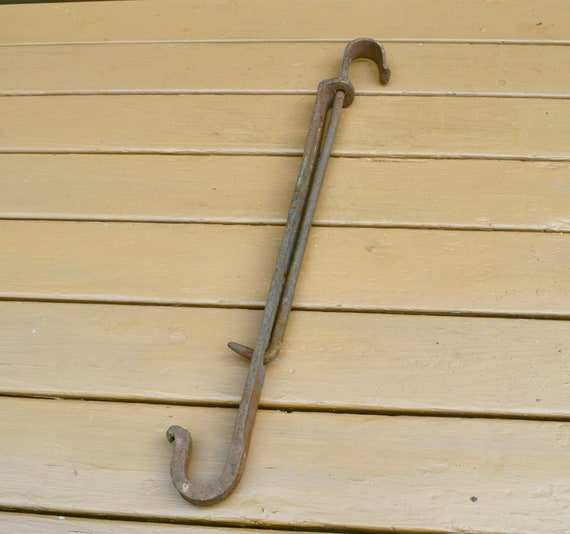The image depicts a pair of intertwined metallic hooks lying flat on a yellow-painted wooden deck. The primary hook is a large, rusted metal piece, with colors blending between red and gray, indicating significant wear. The secondary hook fits through a hole in the primary hook, curving at the top and ending in a sharp point that fits through another hole, suggesting it might be adjustable or extendable. The wooden deck, composed of smooth panels, forms the background, its yellow paint somewhat worn, adding to the rustic aesthetic of the scene. The purpose of these hooks is unclear, but they appear to be some form of tool, possibly posted for sale on a website.